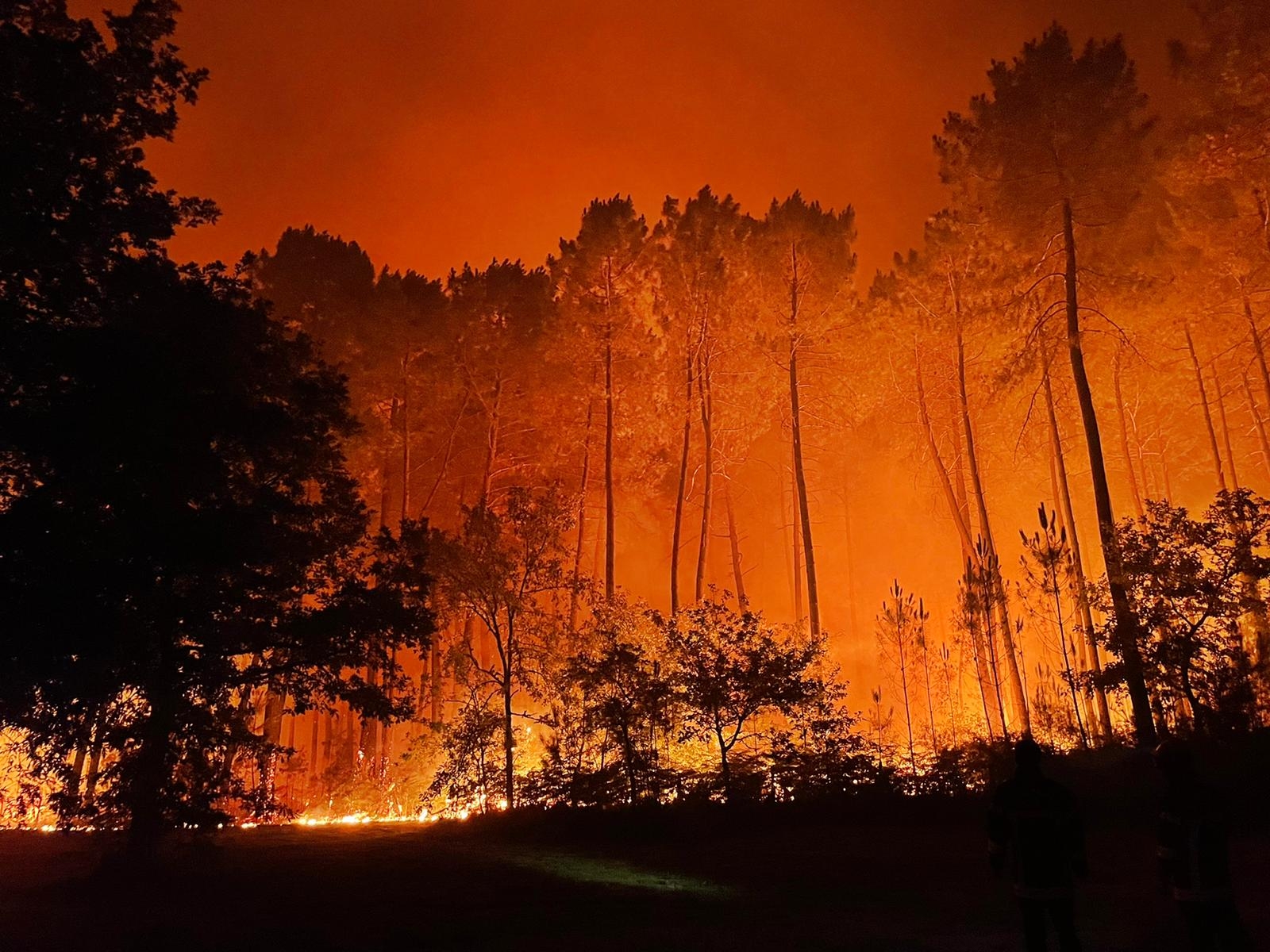The photograph captures a dramatic and intense environment of a forest fire at what appears to be evening or nighttime. In the foreground, the landscape is engulfed in darkness, with the silhouettes of tall, skinny trees standing stark against the glow from behind. The sky above is obscured by thick smoke, blending into hues of orange and brown. A thin line of yellow fire stretches across the landscape, though it is partly obscured by the dense smoke. Flames, in vivid shades of orange and yellow, gradually consume the trees in the background. The distant trees are nearly engulfed, while the ones closer still stand untouched by the advancing inferno. The entire scene is a haunting portrayal of nature ravaged by fire, with an eerie interplay of light and shadow, and the ever-present hint of smoke cloaking the landscape.